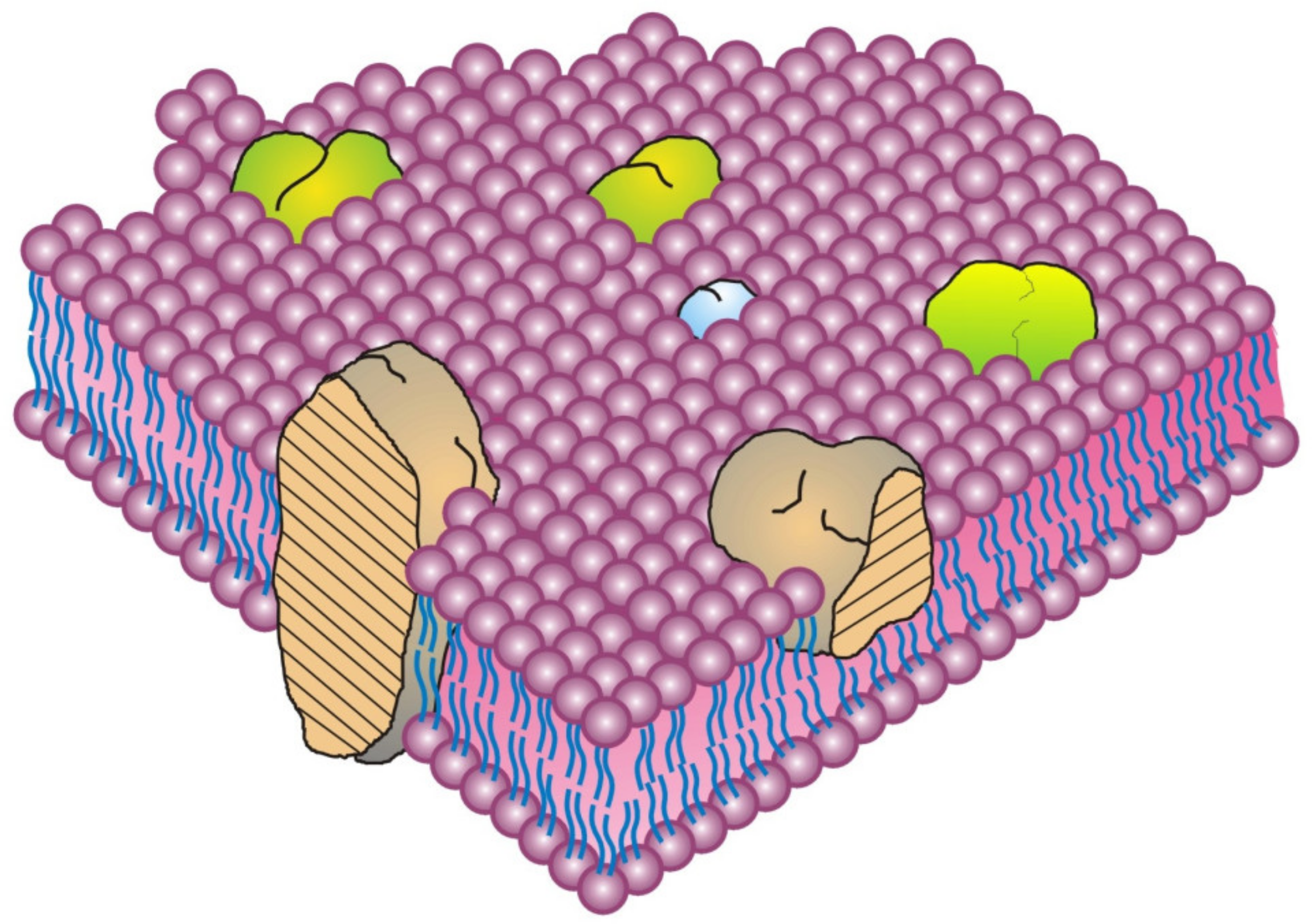The image depicts a detailed, digitally illustrated cross-section of a lipid bilayer, featuring a cartoonish yet three-dimensional quality. From a top-down perspective, we observe layers of pink spherical structures forming a square-like arrangement. These spheres represent lipid molecules, and blue lines extend from them, indicating molecular interactions. Green protruding structures can be seen emerging from among these lipid molecules.

Towards the left side of the image, a large brown, rock-like formation intersects the lipid layer from top to bottom, resembling the bottom of a shoe. On the right side, another similar formation extends from the top to the middle. These formations are likely proteins or other larger molecular complexes embedded within the bilayer.

In the middle of the lipid spheres, there are chunky clusters in shades of green, blue, beige, and yellow, adding to the complexity of the structure. One distinct blue structure stands out prominently amid the pink spheres. Overall, this intricate illustration seems to represent the layers and interactions within a biological membrane, resembling a mix between a scientific diagram and a whimsical ball pit environment.